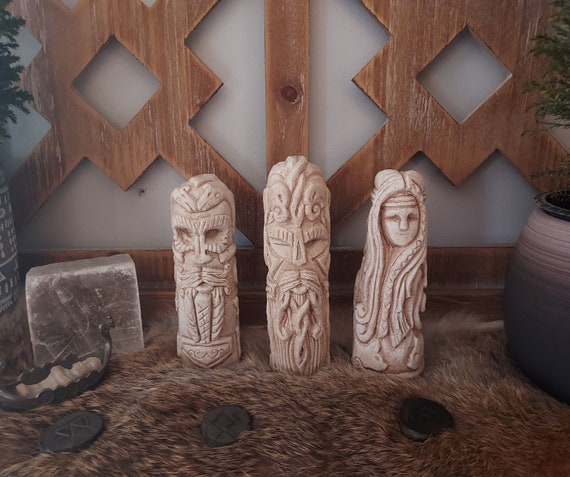In this photograph, we observe a detailed and intricate arrangement set against a gray wall with an elaborate wooden panel featuring a lattice design of diamonds and lines, creating a visually arresting backdrop. Central to the image are three cylindrical Nordic statues, seemingly carved from ivory or stone, displayed atop a fur rug that is brown and white, possibly deer skin. The statues depict two elderly male figures adorned with Viking helmets and braided beards, and to the right, a female figure with long braided hair and a headband. Flanking these figures is a small Viking canoe sculpture made from metal, and in front of the statues are three black circular stones, possibly adorned with carved beads and fish motifs. Additional elements include a pottery planter with green plants situated to the right, another similar planter barely visible to the left, a rock, and three coins placed on the fur. The scene is completed by a rough-edged piece of marble positioned behind the statues and the canoe, adding a touch of rustic elegance to this mantelpiece setting.